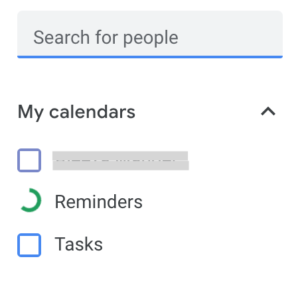The image displays a simplistic and straightforward interface, predominantly white in color. On the left side, there is a grey textbox labeled "Search for People," which is underlined in blue, indicating an active or clickable search function. Below that, the label "My Calendars" is present, accompanied by an upward-pointing arrow suggesting an expandable or interactive feature. 

Next to it, within a purple box, is another component, possibly representing a different calendar or category, bordered in gray. To the right of this, there's a partially visible green "C," which corresponds to an area designated for "Reminders." Lastly, the interface includes a blue box labeled "Tasks." 

The clean and uncluttered layout suggests it could belong to a mobile device, a tablet, or be part of a web page—likely situated as a vertical sidebar for organizational tools. The exact context or platform is unclear from the image alone.